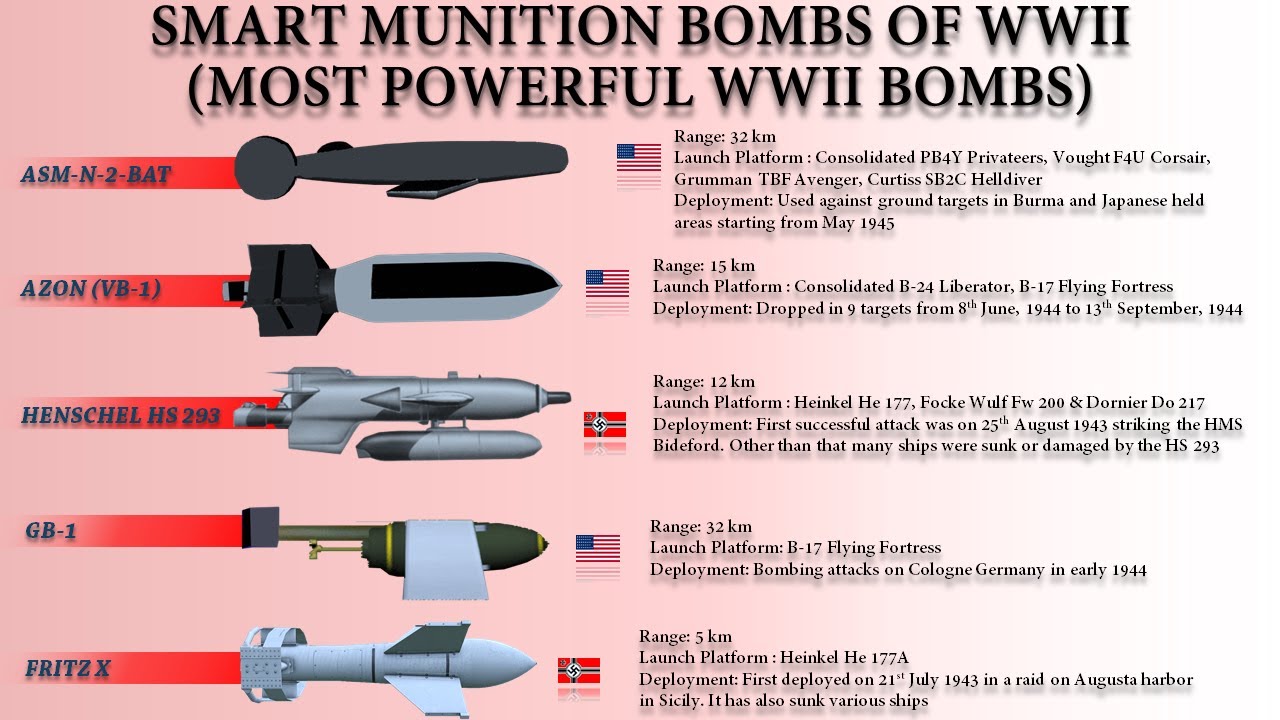The image is a detailed graphic print titled "Smart Munition Bombs of World War II (Most Powerful WWII Bombs)" displayed on a pink gradient background, transitioning from darker pink on the left to lighter pink on the right. The print features five bombs, each with a comprehensive description, a corresponding national flag, and deployment details. The bombs are:

1. **AASM-N-2 RAT**: Depicted as a black or gray cylinder with a rounded nose and wings, accompanied by an American flag. It has a range of 32 kilometers and is deployed from large platforms such as the Consolidated PB-4Y Privateer, Voight F4U Corsair, Grumman TBF Avenger, and Curtis SB-2C Helldiver. It was used against ground targets in Burma and Japanese-held areas starting from May 1945.

2. **AZON VB-1**: Illustrated as a gray and black bomb with a tapered nose and fins in the back, alongside a U.S. flag. It has a range of 15 kilometers and is dropped from large platforms like the Consolidated B-24 Liberator and B-17 Flying Fortress. Its deployment spanned from June 8, 1944, to September 13, 1944, targeting nine locations.

3. **Henschel HS 293**: This bomb looks like a self-propelled rocket with a jet at the back and a snub nose, portraying a Nazi flag. It has a 12-kilometer range and is launched from large platforms such as the Heinkel H-177, Focke-Wulf Fw 200, and Dornier Do-217. The HS 293 was first successfully used on August 25, 1943, against HMS Biddeford, sinking or damaging many ships thereafter.

4. **GB-1**: Shown as a cylindrical body with a tapered nose and a thin pole, accompanied by a U.S. flag. It has a 32-kilometer range and is deployed from the B-17 Flying Fortress. It was used in a bombing attack on Cologne, Germany, in early 1944.

5. **Fritz X**: Depicted as a bomb with a tapered nose and two wings, bearing a Nazi flag. It has a range of 5 kilometers and is deployed from the Heinkel H-177A. The Fritz X was first used on July 21, 1943, and notably in an August raid on Augusta Harbor in Sicily.

Each bomb is identified with a red banner to the left of the graphic, and detailed information on range, deployment platform, and initial use is provided to the right of each corresponding illustration and flag.